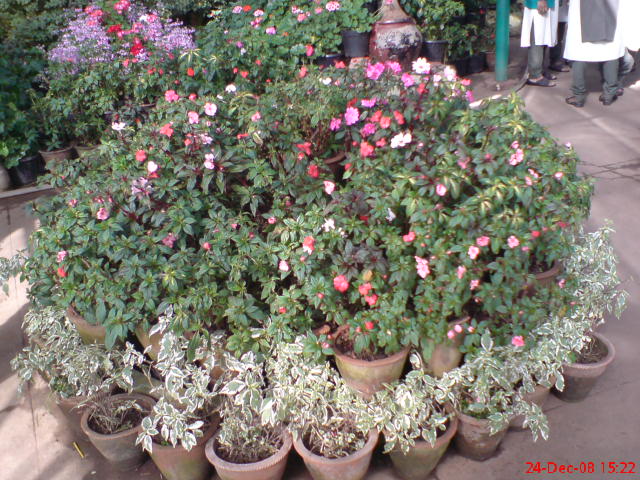This detailed color photograph, seemingly taken at a nursery or garden, features an array of individual flowerpots arranged thoughtfully. In the foreground, several pots brim with vibrant flowers in hues of pink, white, and red. Surrounding these, an outer circle displays plants with silvery green foliage. Beyond this circle, there are additional pots, some containing purple blooms, creating a layered visual effect. In the bottom right corner of the image, the timestamp '24-DEC-08, 1522' is visible in red. The green plants with just leaves lie below a road, enhancing the contrast with the floral arrangements. The lower halves of two individuals are seen near a teal-greenish pole, one wearing gray pants and a knee-length white jacket, while the other sports a long jacket that is teal on top and white at the bottom. The flowerpots, mostly brown and sooty with some black ones in the background, form a structured and circular arrangement, adding to the overall symmetry and organized beauty of the scene.